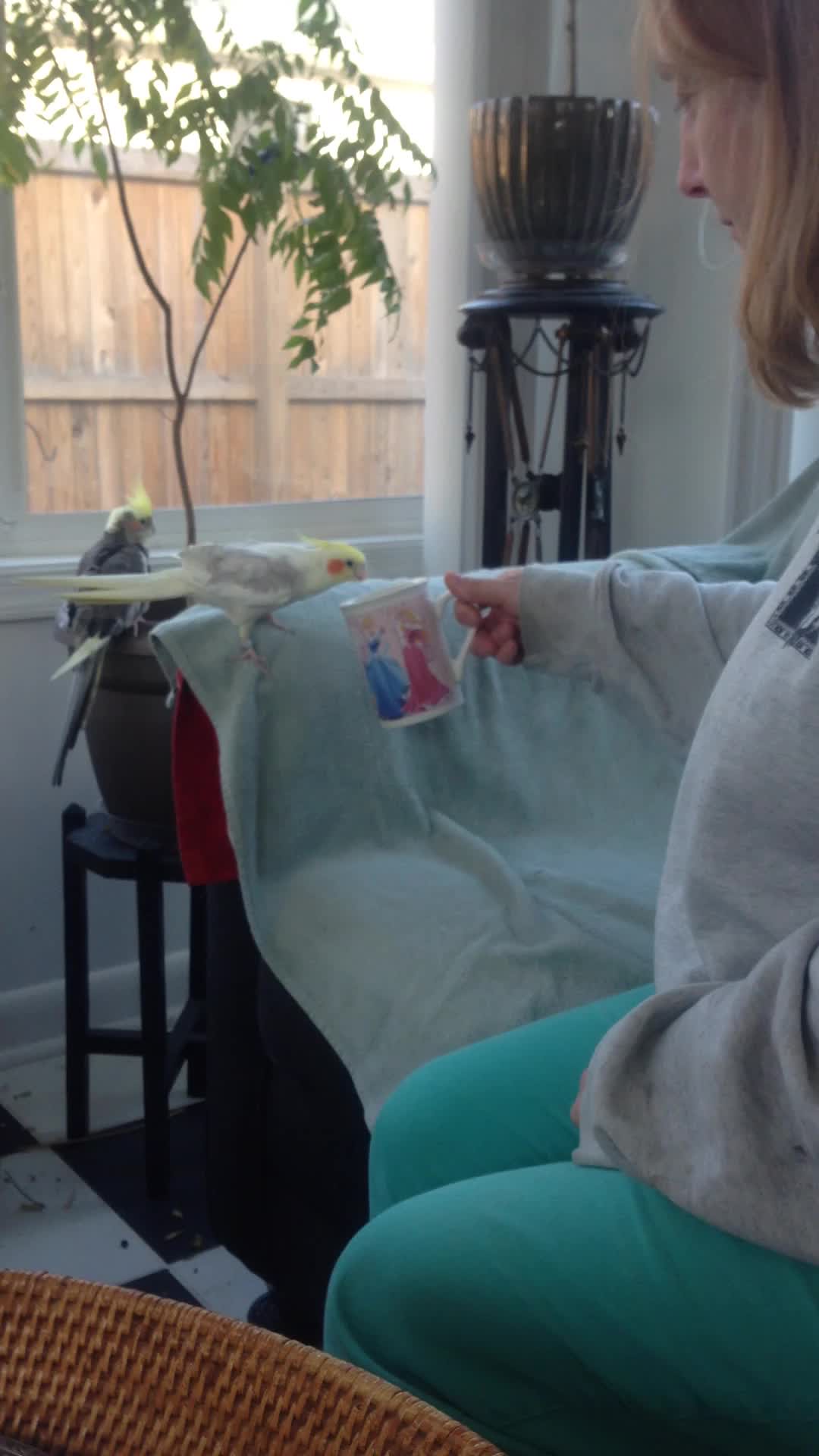In this detailed photograph, a woman wearing green pants and a long-sleeved grey sweatshirt sits on the right side, her long blonde hair cascading down as she holds out a white mug adorned with Disney princesses. She appears to be offering something to a parakeet, which is perched on the arm of a chair or sofa draped with a towel. This parakeet, prominently featured in the center, has striking grey and white feathers with a vibrant yellow and orange head. Nearby, another parakeet, darker in color with yellow on its top, stands on the pot of a potted plant, gazing out through a single-paned window. The window, framed in white, reveals an outdoor scene of a brown plank fence and a white wall beyond it. The room’s floor is a black and white checkerboard tile, providing a stark contrast to the wicker furniture edge seen in the foreground. A tall, round, shell-textured black vase sits atop a long side table in the back corner, adding a decorative touch to the interior. The walls of the room are white, and in the upper right corner, there is a dark brown pedestal-like stand or lamp.